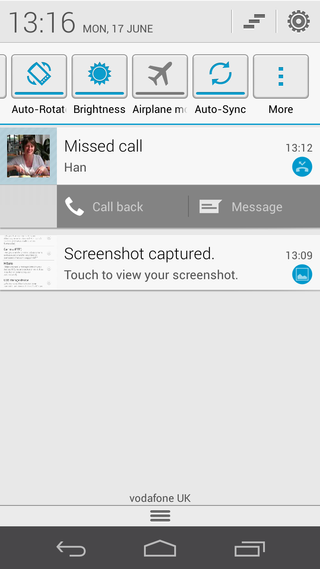The image showcases a screenshot from a mobile device's interface. 

In the upper left corner, the time is displayed as 13:16. Next to it, the date is indicated as MON 17th June. The settings icon, shaped like a wheel, is positioned in the upper right corner.

The main section of the interface features several icons and labels. First is the image of a blue cell phone, followed by "Auto Rotate." Below this is an icon resembling a blue sun, labeled "Brightness." An airplane icon in gray is displayed beneath, with "Airplane Mode" next to it. Further down, two arrows forming a circle indicate "Auto Sync," followed by an ellipsis (three small dots) labeled "More."

A notification section beneath shows an image of a woman with short dark hair, dressed in a white shirt, within a square. Beside her image, the text "Missed Call" is displayed. Underneath her name, abbreviated as "HAN," is a white phone icon labeled "Callback" and a white notebook icon labeled "Message." 

A gray notification indicates "Screenshot captured. Touch to view your screenshot." Below this entry, another time reading 13:09 is visible, alongside a blue circle with an icon resembling a laptop screen inside it.

At the bottom of the interface, "Vodafone UK" is written in gray text.